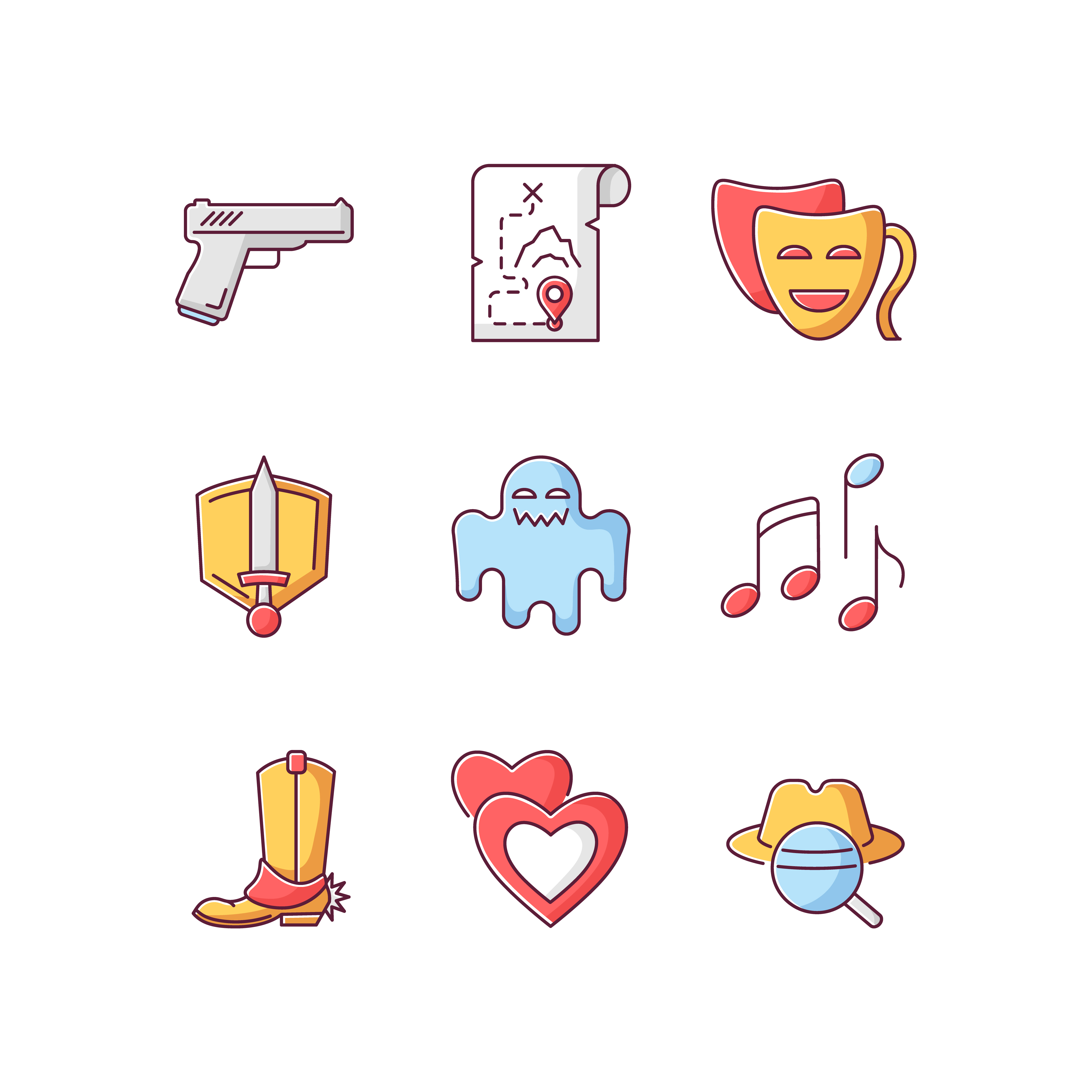The image appears to be a collection of nine cartoonish, round-edged icons arranged in a tidy 3x3 grid, resembling emojis or an icon pack. The top row features a light gray handgun on the far left, a detailed treasure map with a trail leading up a mountain and a Google postmark in the middle, and a golden, smiling theater mask on the right. The middle row includes a golden shield with a gray sword in front of it on the left, a light blue ghost with a spooky face in the center, and a set of colorful musical notes to the right—a pair of downward red notes beside an upward blue note. The bottom row starts with a yellow leather cowboy boot on the left, followed by two hearts in the center—one solid red, the other red outlined with a missing centerpiece—and finishes with a yellow detective hat positioned behind a magnifying glass on the right. The icons exhibit a consistent color scheme dominated by light red and mustard yellow hues.